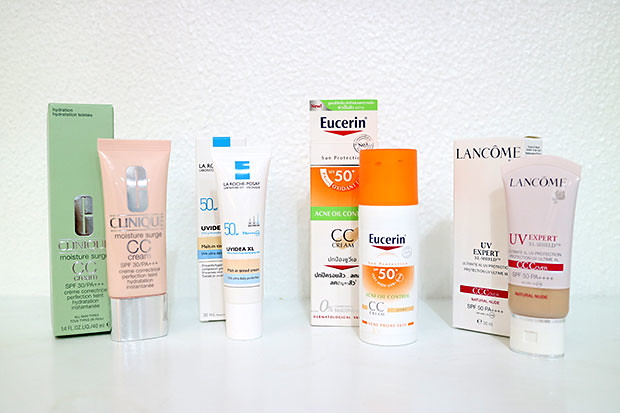The image features a white-walled background and a table that is adorned with various cosmetic products. On the left side of the table, there is a green rectangular box with a 'C' logo, which appears to be a moisture-related product. Next to it, there is a tube of clinic cream labeled 'CC'. This tube has a predominantly pink design with a silver base and a pink cap.

Further to the right, there is a white bottle of Eucerin, distinguished by an orange segment in the middle and the brand name prominently displayed. Additionally, there is a Lancome product; this is a white bottle featuring a beige middle layer and a white cap. The entire arrangement is presented on a white table against the white wall, creating a clean and crisp visual composition.